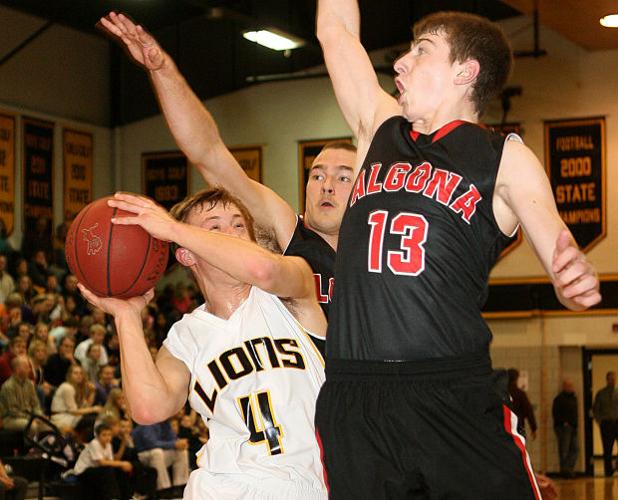In an indoor gymnasium packed with spectators, a high-intensity basketball game unfolds. In the foreground, a young player in a white Lions uniform, numbered four, tightly grips the basketball with both hands, searching for an opportunity to pass or shoot. He appears focused yet guarded, as he is closely marked by two defenders from the opposing team, Algona. One of these defenders, wearing a black jersey with red accents and the number 13, is captured in mid-air with an arm outstretched, attempting to block the pass or shot. Another Algona teammate is also seen, arm extended, adding to the defensive pressure. The dynamic scene is sharply in focus, emphasizing the tense moment, while the background shows a crowd of blurred onlookers and wall decorations, including a banner that reads "Football 2000 State," indicating the gym's multi-sport usage, most likely in a high school setting. The players, possibly teenagers or in their early twenties, exhibit a mix of determination and athleticism typical of competitive youth sports.